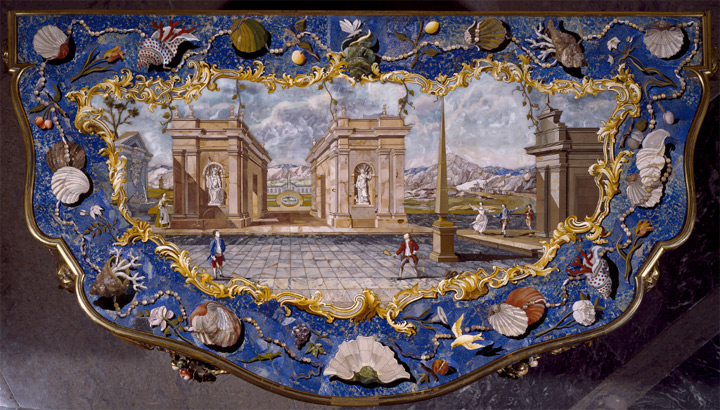The image depicts an intricately framed painting set against a grayish bronze background. The ornate frame is gold with elaborate, wavy edges that transition into a rounded bottom, accentuating its distinctive shape. Surrounding the painting is a decorative border composed of an array of multicolored seashells—white, gray, red, and yellow—interconnected by delicate chains of beads or tiny shells. These shells and beads are set against a bright blue background interspersed with beige and tan spots. Inside this ornate frame lies a vivid scene featuring two men dressed in old-fashioned costumes, poised to duel or engage in a game. They stand on a rock-finished ground in a courtyard, flanked by spectators on the right. The backdrop includes grand, gray stone buildings with columns and towering statues, evoking a sense of historical grandeur.